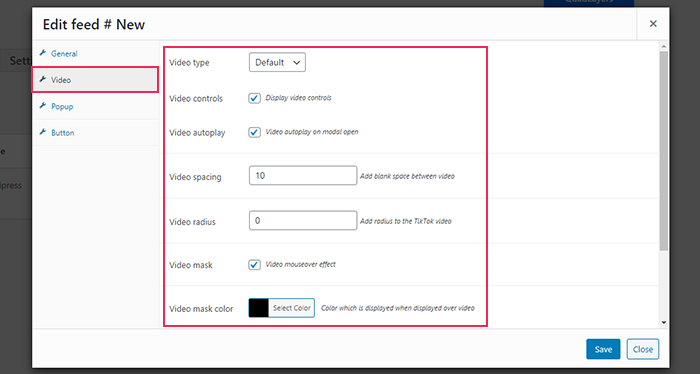The image features an "Edit Feed" interface, indicated by the text "edit feed #new" at the top, highlighted with a light gray line running horizontally beneath it from left to right. This interface includes four navigational items listed in blue text: "General," "Video," "Pop-up," and "Button." 

Among these, "Video" is emphasized with a red rectangular box around it. To the right of this, there is another red rectangular box enclosing an array of video settings and options. 

Inside this red box, the following features are visible:
- A label "Video Type" with a drop-down menu set to "Default."
- "Video Controls" accompanied by a checkbox that is marked with a blue check, indicating that display video controls are enabled.
- "Video Autoplay" with a similarly checked box, specifying "Video autoplay on modal open."
- Underneath this, the text "Video Space" followed by "10" along with instructions to "Add blank space between video."
- "Video Radius" set to "0," with a note to "Add radius to the TikTok video."
- "Video Mask" alongside a checkbox with a blue check, denoting that the video mask feature is activated.
- Lastly, it mentions "Video Mouse Over Effect," suggesting additional settings available for managing the video's mouse-over functionality.

The organized layout of settings within the red rectangular box indicates a comprehensive feature set designed for detailed video customization in the interface.